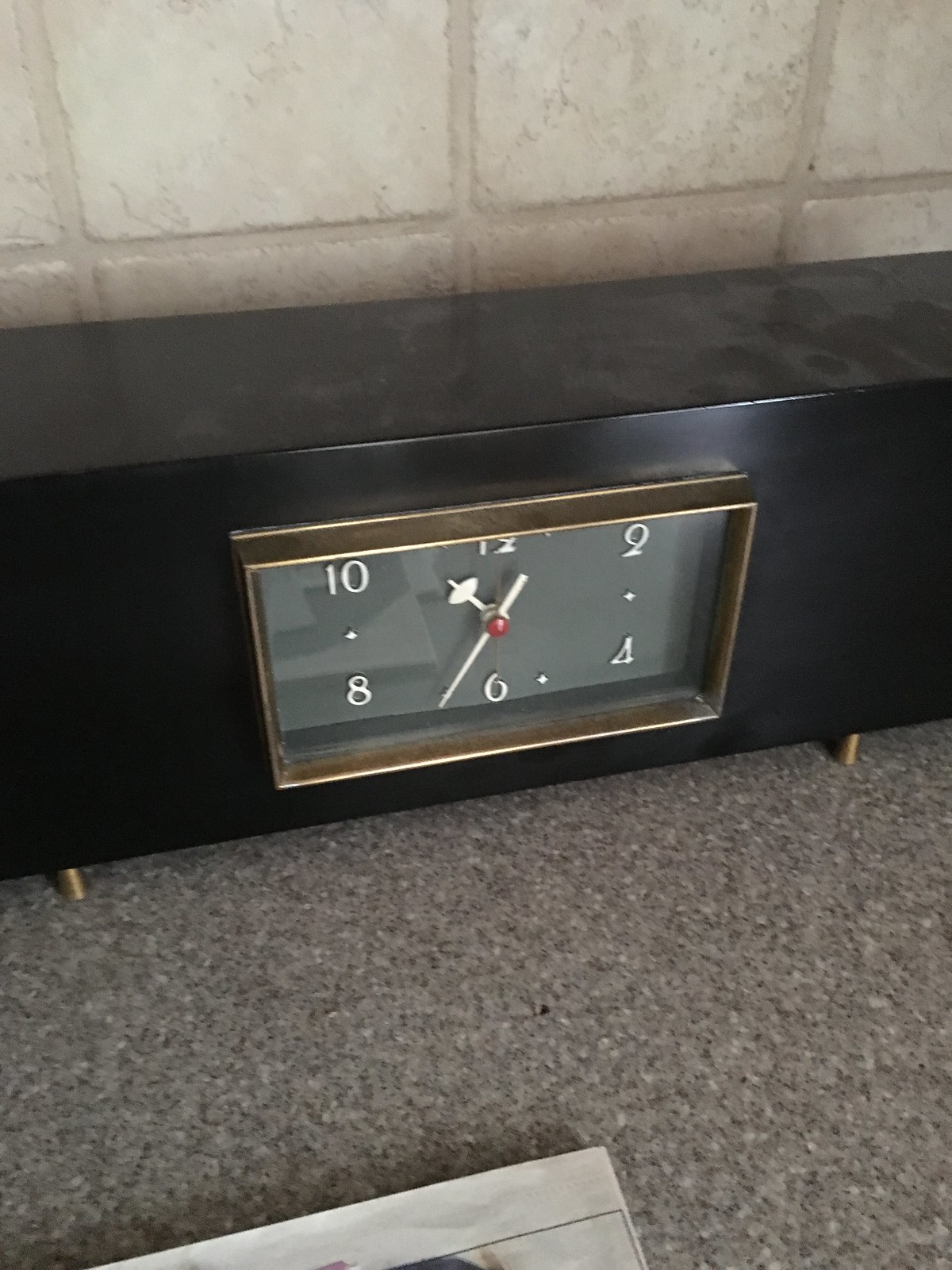A black, rectangular clock with gold feet and a gold-trimmed face sits elegantly on a gray granite kitchen countertop, displaying the time as 11:30. The beige tile backsplash provides a warm and neutral background, enhancing the sophisticated appearance of the clock. In the bottom corner of the image, a newspaper is casually placed on the countertop, adding a touch of everyday life to the scene. The photograph is meticulously composed, focusing primarily on the clock, countertop, and backsplash, capturing the essence of a serene and stylish kitchen setting.